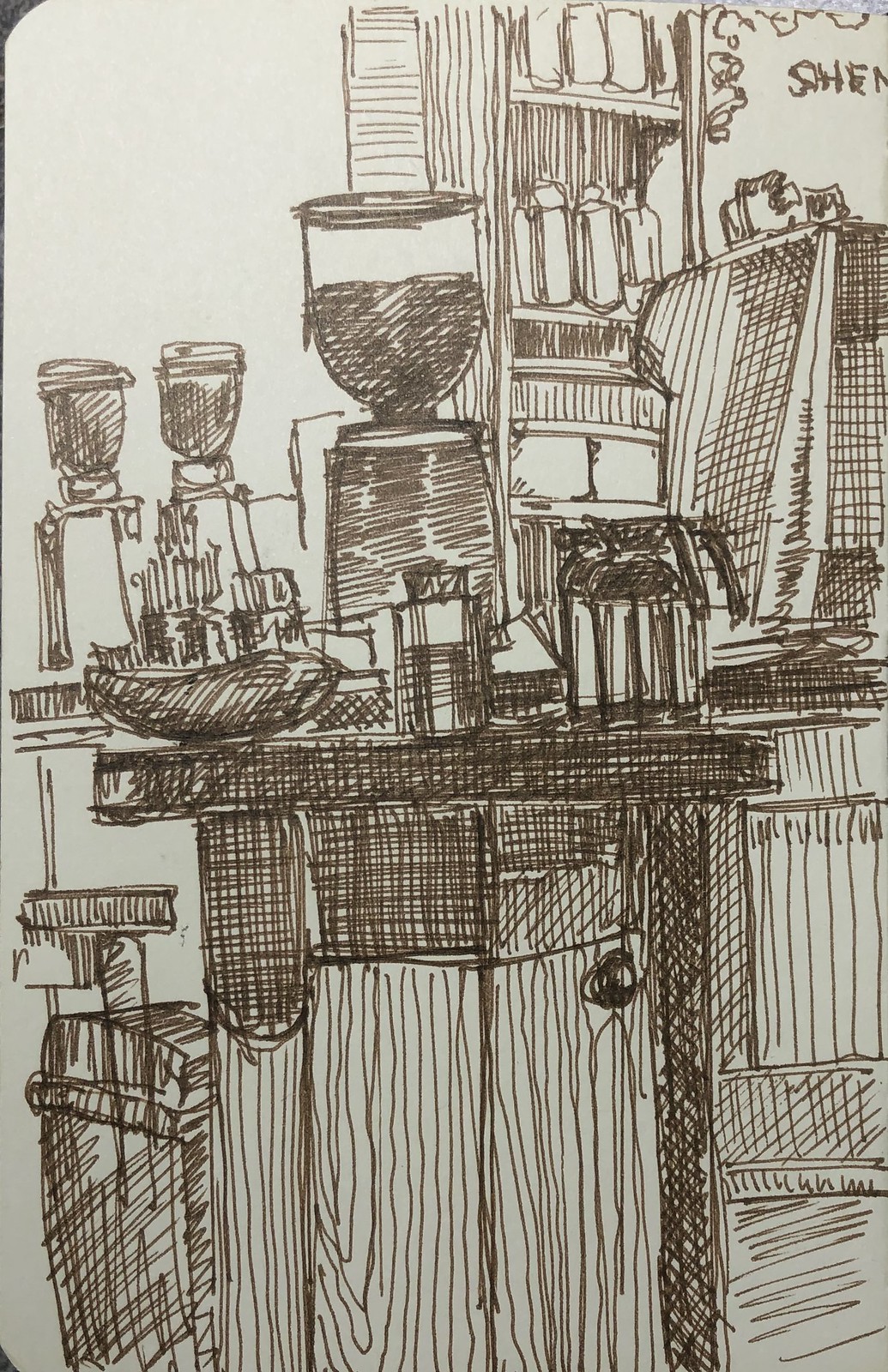This detailed black and white pen and ink sketch features a central large blender with dark contents, flanked by two smaller blenders in the background, all atop a wooden cabinet with a single door and a knob. Adjacent to the main blender are a couple of old-fashioned coffee pots. The blenders and coffee pots rest on the cabinet's rectangular surface, which also accommodates an oblong dish and a round basket holding square, dark objects. In the background, a second surface with two additional blenders and a shelving unit holding jars, bottles, and possibly cartons of milk is visible. The shelf also features a pot and a hook with hanging objects, beneath which a towel is draped. The overall grayish cream paper background enhances the dark brown ink, with the shading and intricate lines adding depth and texture. The top right corner of the sketch includes partially visible letters "S-H-E-N," hinting at an incomplete word. The setting resembles a café or a kitchen, filled with various containers and utensils, evoking a sense of everyday bustle and organized clutter.